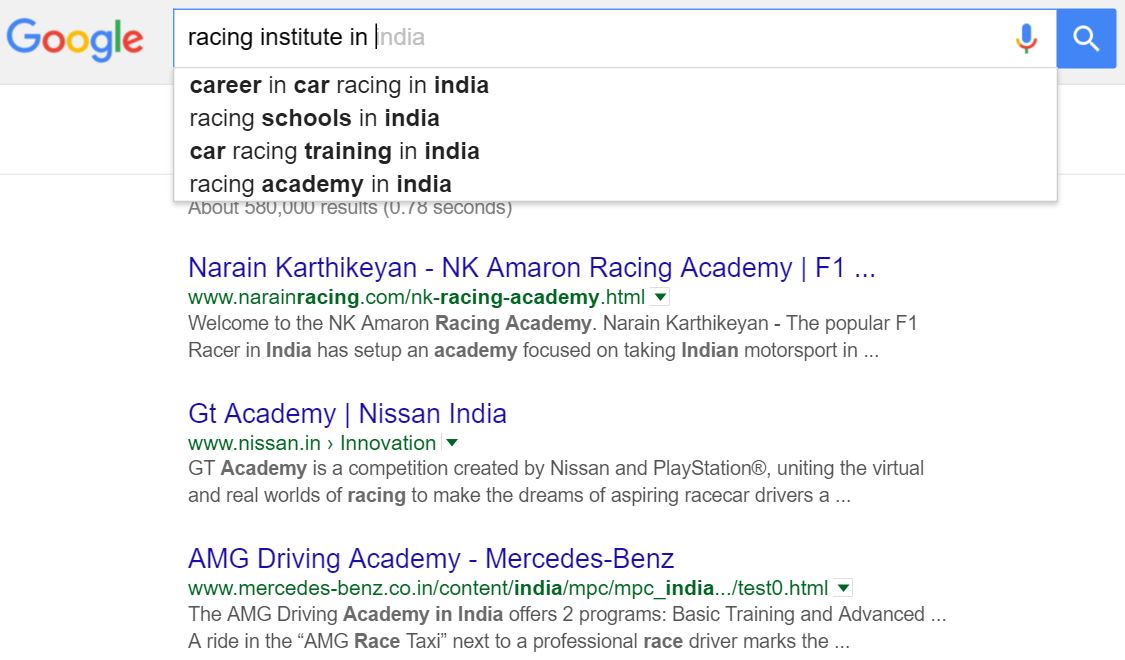A screenshot captured from a Google search, showcasing the query "Racing Institute." The autocomplete function suggests "India" as the next term, likely indicating that the user is either currently in India or frequently searches for India-related topics. The search results indicate approximately 580,000 entries, generated in 0.78 seconds. 

The first search result is linked to the Narain Karthikeyan or NK Racing Academy, associated with Formula 1. The second result points to the GT Academy by Nissan in India. The third result refers to the AMG Driving Academy by Mercedes-Benz, highlighting that the academy offers two programs: Basic Training and Advanced Training. Additionally, it mentions that a ride in the AMG Race Taxi with a professional race driver concludes the experience.

The screenshot primarily displays the search results within the Google search bar. Other details such as the device used or the time the screenshot was taken are not visible, although the layout suggests it was likely captured on a laptop. The background of the screenshot is predominantly white.